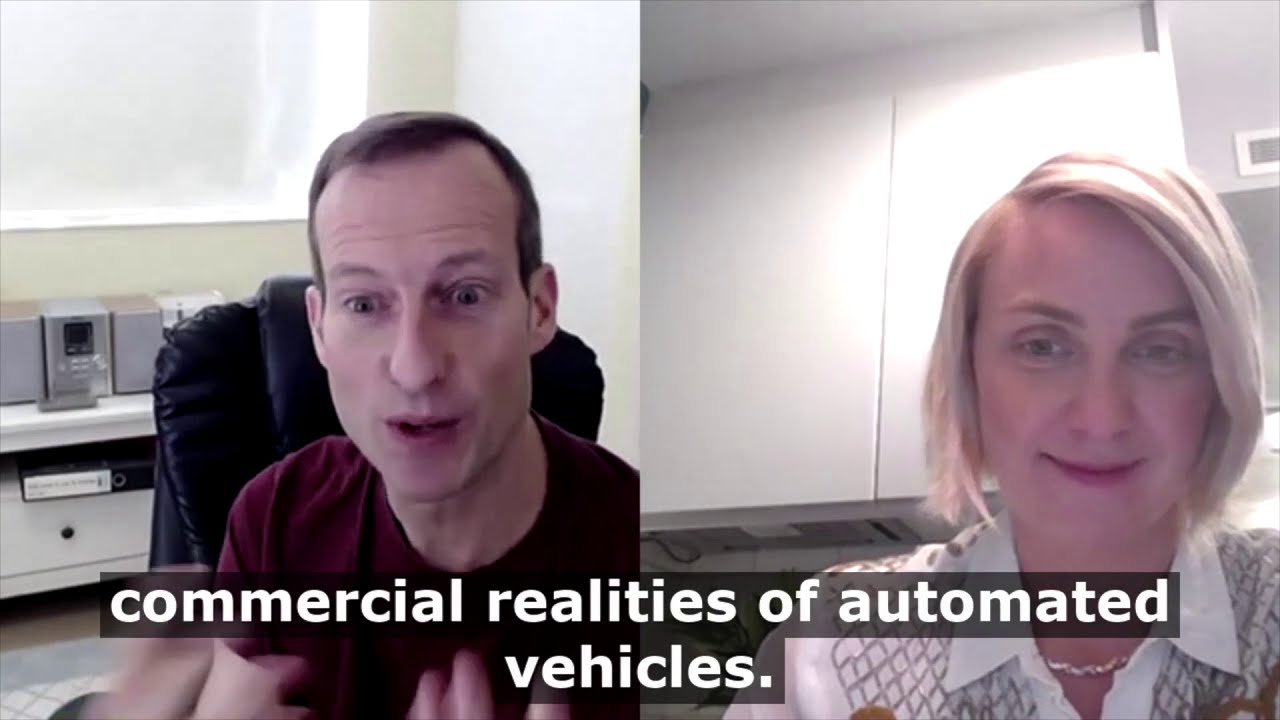The image is a screen capture from a video call featuring two Caucasian individuals, split down the middle. On the left side is a middle-aged man with brown hair, wearing a red short-sleeved shirt, and seated in a black computer or office chair. The background reveals a white wall with a small stereo system sitting on a white table. His hands are slightly raised in front of him, and his mouth is slightly open as though mid-conversation.

On the right side is a nicely dressed woman with medium-length bleached blonde hair and brown eyebrows, complimented by thin red lips. She is wearing a white blouse with a silver-toned checkered pattern and a gold necklace. The background shows white cabinets and an air duct. She is smiling, looking engaged, possibly listening to the man on the left. The text at the bottom of the image reads “Commercial Realities of Automated Vehicles” in white letters with a black border.